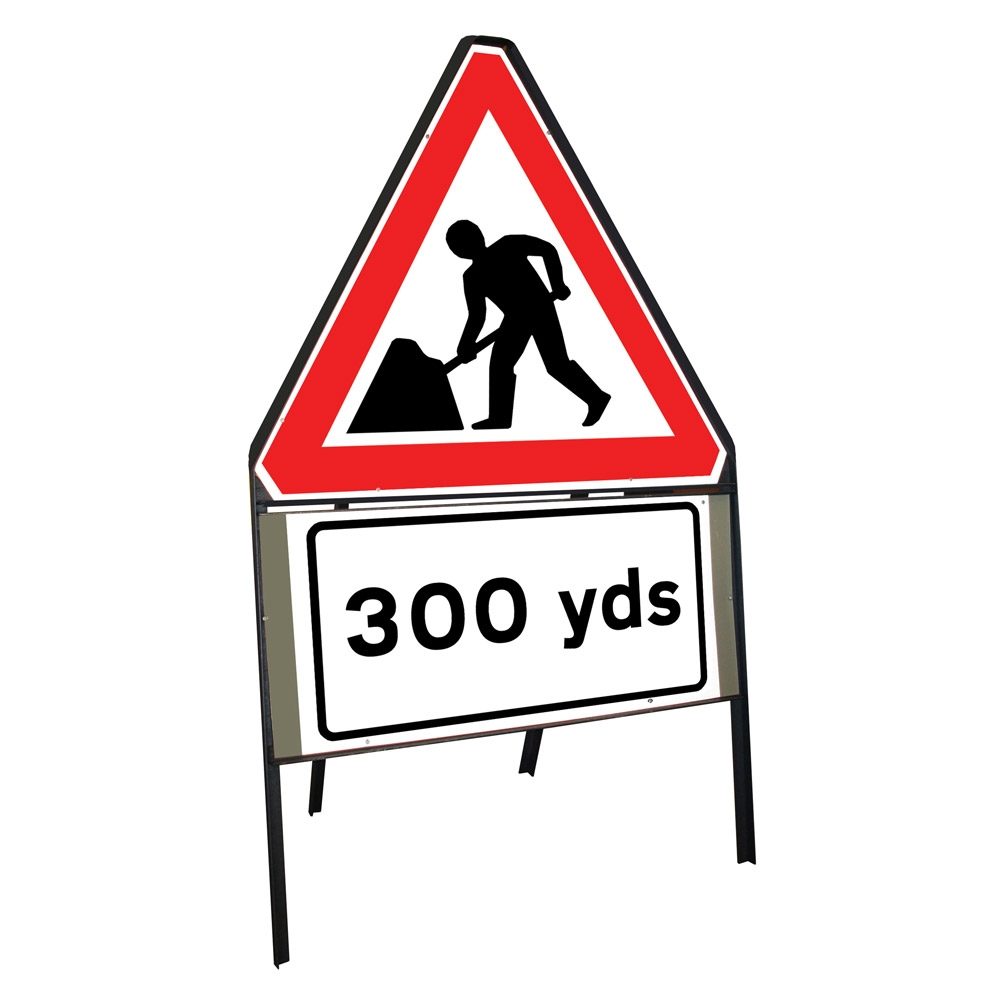This image is a 3D rendering of a roadway sign designed to be freestanding on four dark gray legs. The sign features two distinct sections. The top section is a triangular sign with a red border enclosing a smaller white triangle, within which there is a black silhouette of a man shoveling into a black dirt mound. This triangular sign is indicative of roadwork ahead. Directly below the triangle is a rectangular white sign bordered in black with rounded corners, containing black text that reads "300 YDS," denoting the distance to the roadwork. The front two legs that support the sign are clearly visible, while the back two legs are partially obscured.